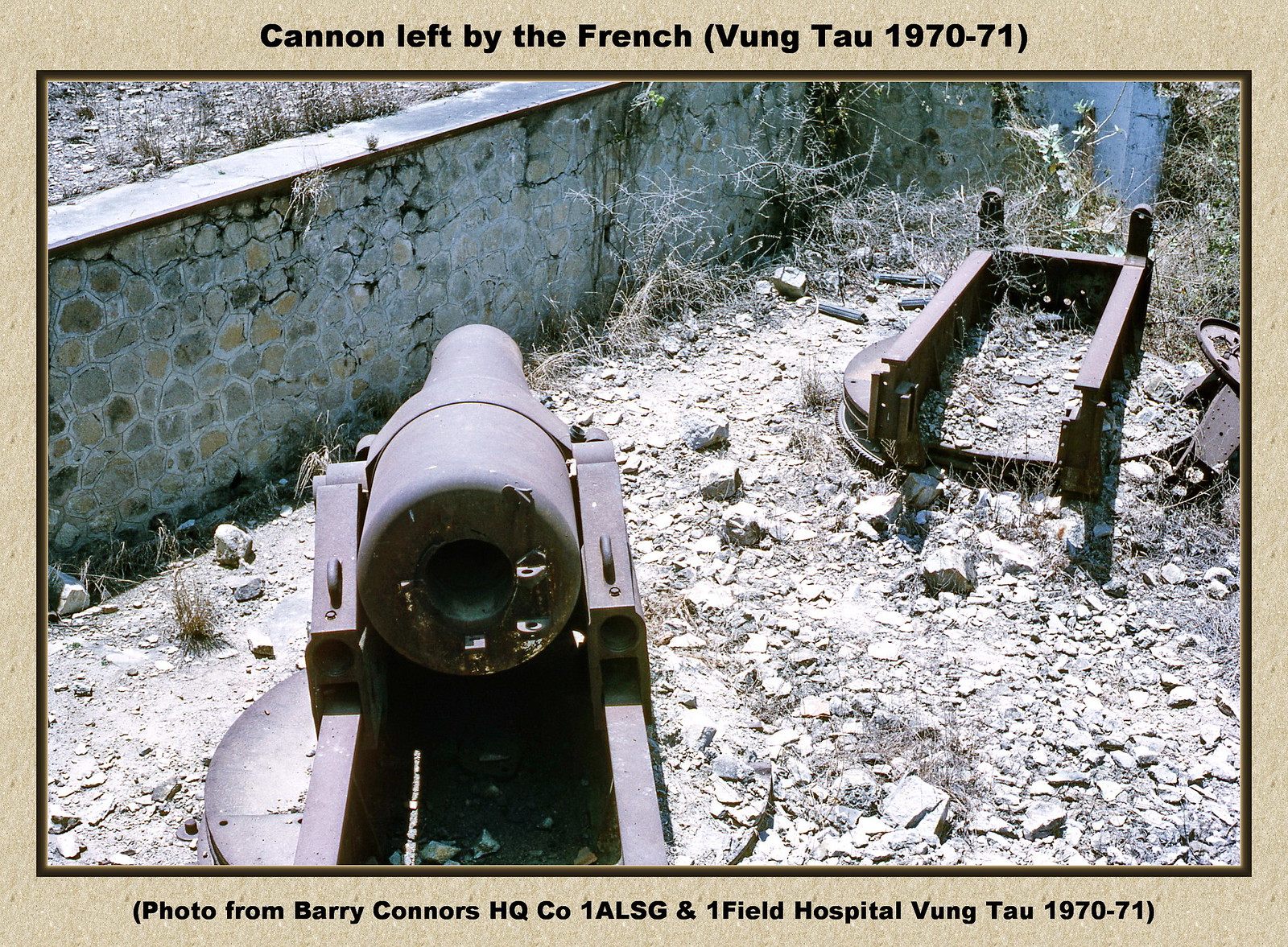The image depicts a vintage outdoor scene from daytime, framed with a brown or tan border that resembles construction paper with visible fibers. Dominating the foreground is a rusted, brown steel cannon left by the French, presumably during the years 1970-1971 in Vung Tau. The cannon is grounded and detached from its base, with an empty, likely damaged metal square base located to its right, showing disconnected bolts. The scene is littered with debris, featuring an array of large and small rocks, alongside pieces of rusty metal and dry brush scattered across the dirt-laden ground. A decaying brick retaining wall, partially crumbled at the top, stands amidst this rubble. Black text at the top of the image reads, "Cannon left by the French, Vung Tau 1970-71," while the bottom caption states, "Photo from Barry Connors HQ, CO1, ALSG and Onefield Hospital, Vung Tau 1970-71."